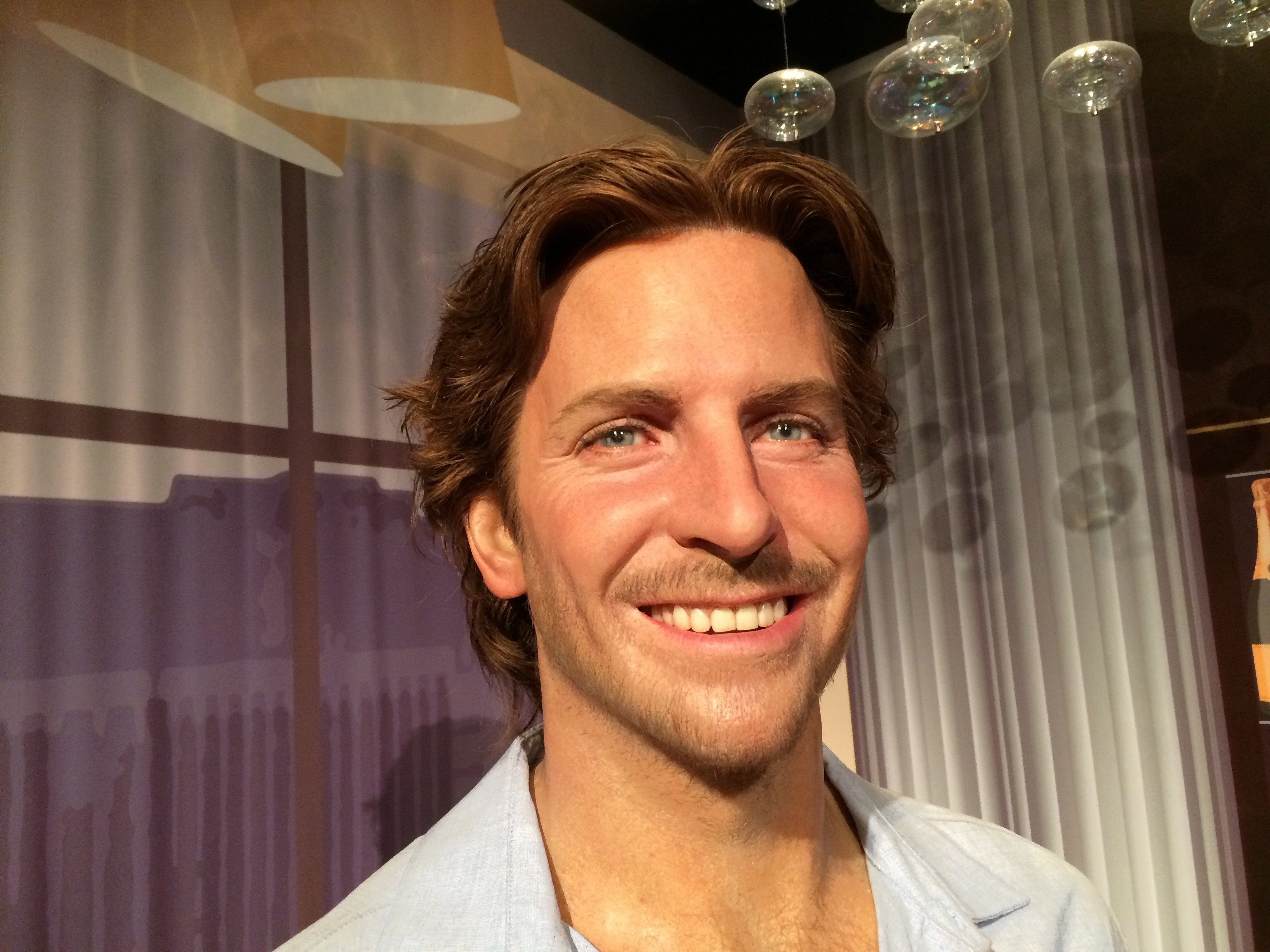This is a detailed close-up photograph of actor Bradley Cooper, taken in a landscape orientation. The image prominently features his smiling face and shoulder area. Bradley, a white man with blue eyes and brown hair, is captured in mid-smile, showcasing his straight white teeth. He is wearing a white blazer over what appears to be a light blue shirt. In the background, there are decorative elements, including a purplish curtain with a building-like design on his right and a plain white curtain on his left. Above him, several glass globes, resembling hanging bubbles or chandelier spheres, are visible. The image is set in a room that possibly resembles a stage or a styled interior space.